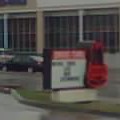This tiny photo, smaller than a postage stamp, requires close inspection to discern its details. At the forefront of the image is a white, changeable letter sign with a red header, typically seen on roadsides, laying on the ground just beneath a grassy embankment. The sign features black lettering, though the text is indiscernible. In the background, a car is parked in what appears to be a parking lot, adding context to the scene. Further beyond, a building with numerous windows and distinctive white columns looms, providing a backdrop that juxtaposes the simplicity of the sign against a structured architectural setting.